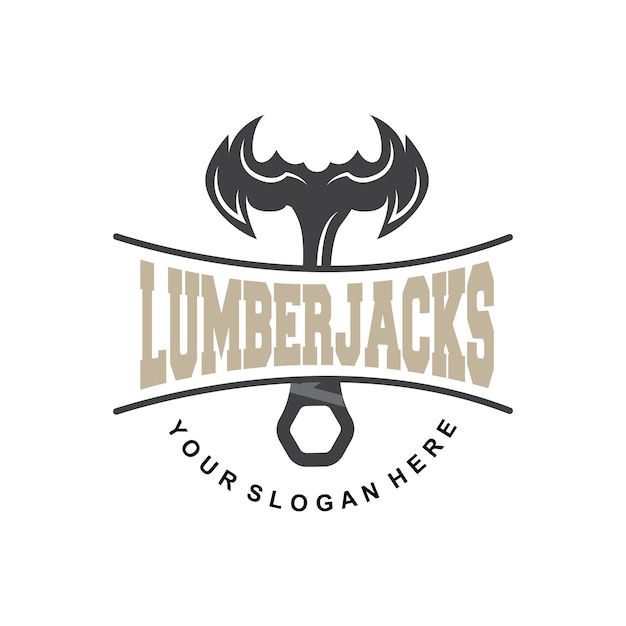The image presents a logo set against a white background, likely designed as a web page template. Central to the logo is a stylized, double-sided axe that resembles the Batman symbol, featuring a jagged, black outline with white accents. This distinctive shape is anchored by a handle, giving the appearance of a tool in profile. At the heart of the axe, in light brown text, is the brand name "Lumberjacks," flanked by identical black curved lines above and below it. Beneath this, there's a hexagon shape, suggesting the end of a bolt or a nut. The entire design is sleek and modern, and under the hexagon, the phrase "YOUR SLOGAN HERE" is displayed in bold, black, capitalized letters, providing space for customizable branding.